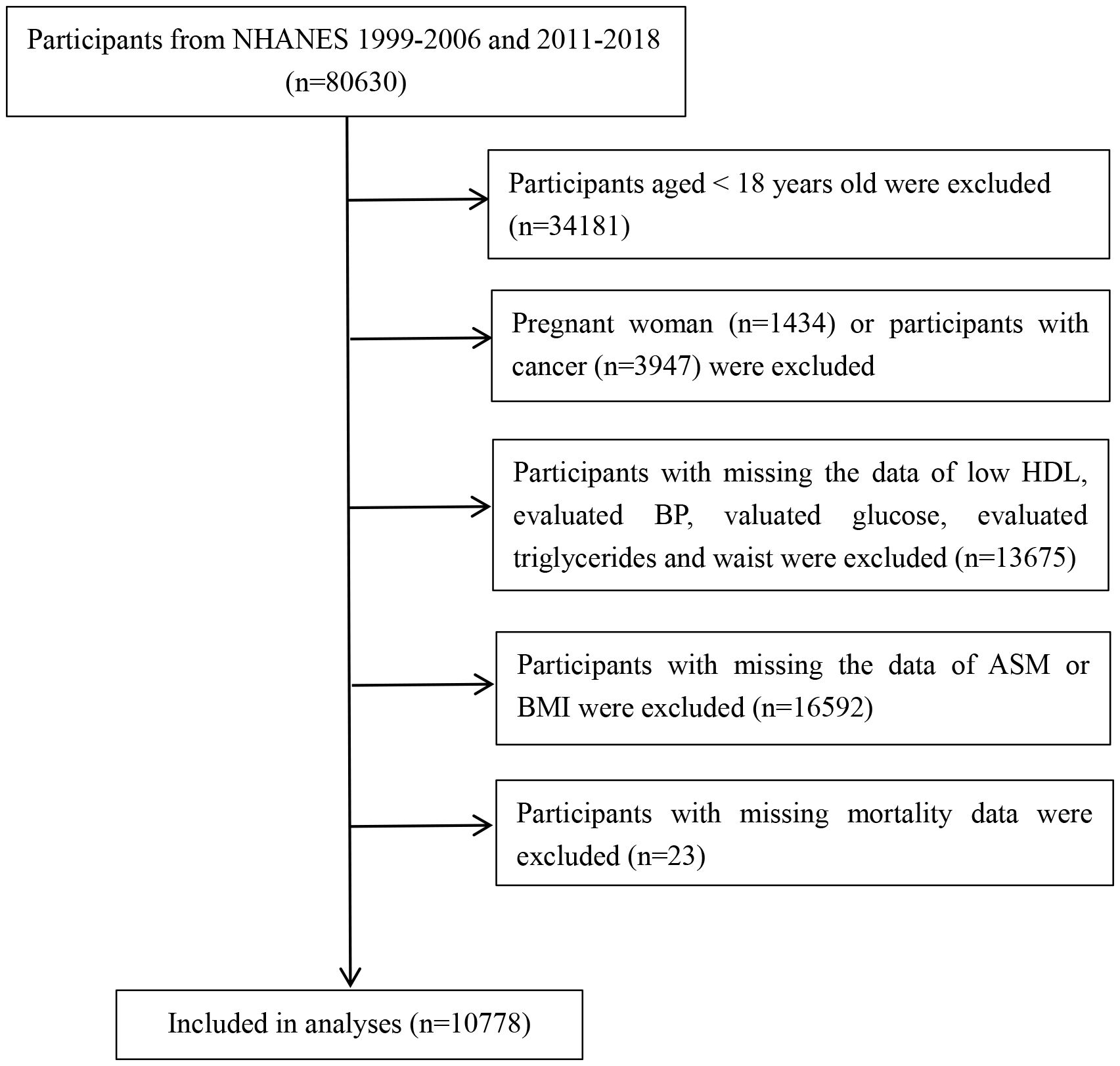The image is a detailed filtering diagram from the NHANES study for the periods 1999-2006 and 2011-2018 with an initial participant pool of 80,630. The process of exclusion is illustrated through a series of boxes and arrows. Participants under 18 years old were excluded first (N=34,181), followed by the exclusion of pregnant women (N=1,434) and those with cancer (N=3,947). Subsequently, participants with missing data on key health metrics - low HDL, evaluated blood pressure (BP), evaluated glucose, evaluated triglycerides, and waist measurements - were excluded (N=13,675). Next, participants missing data on appendicular skeletal muscle mass (ASM) or body mass index (BMI) were excluded (N=16,592). Following that, participants with missing mortality data were excluded (N=23). The final analyzed sample included 10,778 participants.